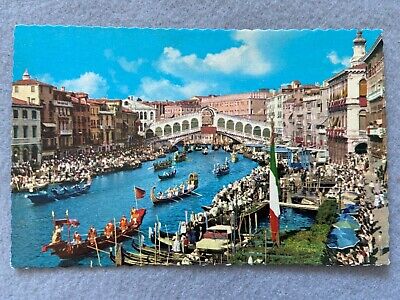This is a vintage, mid-century postcard of the Grand Canal in Venice, Italy, featuring a vibrant and bustling scene. The image, though somewhat blurred, centers on a large, white arched bridge with multiple window-like arches spanning the canal. The canal is filled with several gondolas and other boats, suggesting a lively event, possibly a boat race or a traditional celebration like the blessing of the gondolas. 

At the forefront, a red boat with five people and a red flag leads, followed by a blue boat to its right and a green one further back. Behind them, five more boats are paddling in a similar direction. The canal is lined with many onlookers standing or sitting under umbrellas at cafés, perched on risers, or simply watching from the busy streets and old, colorful buildings that flank the waterway. The surroundings are adorned with the charm of pink and white architecture, contributing to the vibrant atmosphere.

An Italian flag is prominently displayed on a pole in the middle right of the image, reinforcing the Italian setting of this picturesque scene. This reflection of Venice captures the essence of a lively moment, frozen in the enchanting blur of a historical photograph.